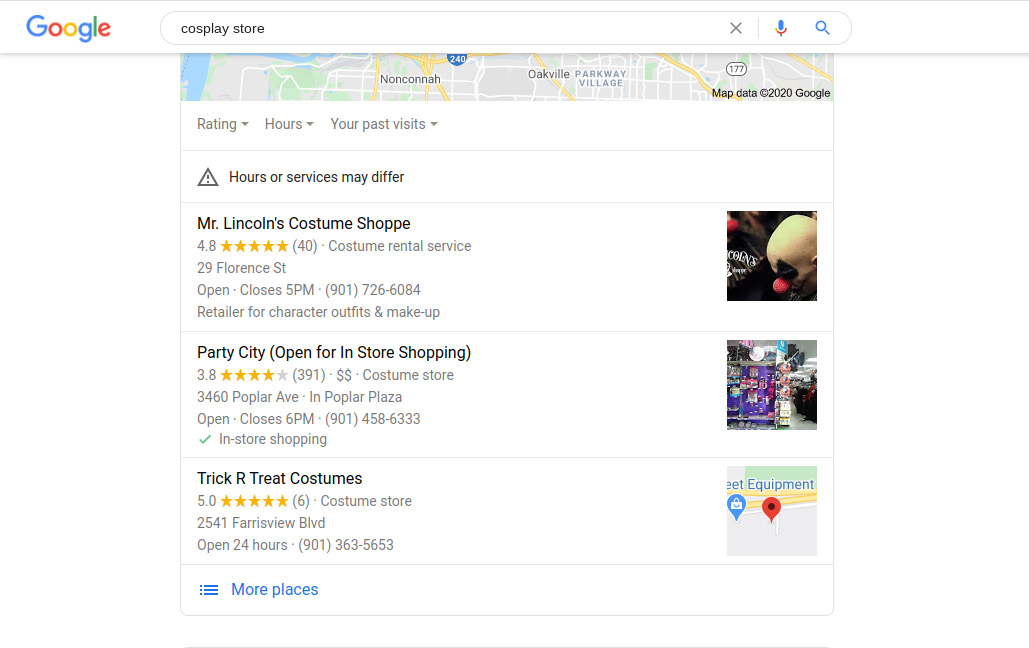A Google search results page showcases various cosplay stores. In the search box, the term "cosplay store" is entered. Below, several listings are displayed. The first listing is for "Mr. Lincoln's Costume Shop," which includes the location, hours of operation, phone number, and a notation about selling character outfits and makeup. This store has a 4.8-star rating out of five and features a photo of a creepy clown with a red nose and bald head.

The second listing is for "Party City," indicating it is open for in-store shopping, with a green checkmark to denote this status. It includes the address, hours of operation, and phone number. This store has a 3.8-star rating out of five and features a small image of the store's interior.

The third listing is for "Trick-or-Treat Costumes," which provides the address, hours of operation, and phone number. This store boasts a perfect 5.0-star rating out of five and is represented by a map image. Each store's name is accompanied by its respective image on the left side of the listing.